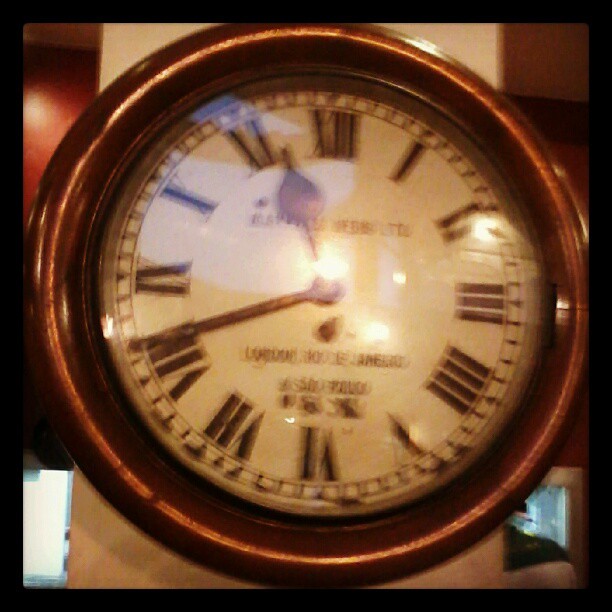This image depicts a slightly blurry round clock with a reddish-brown border, possibly made of wood or metal. The clock face is white and features Roman numerals to indicate the hours. The clock hands are positioned at 11:40. Although there is some writing on the clock face, it is not legible. The background behind the clock is dark brown, while the clock itself appears to be mounted on a light brown board. In the bottom right corner of the image, there is a square area containing blue and black colors. Additionally, a reflection of light can be seen on the glass covering the clock face.